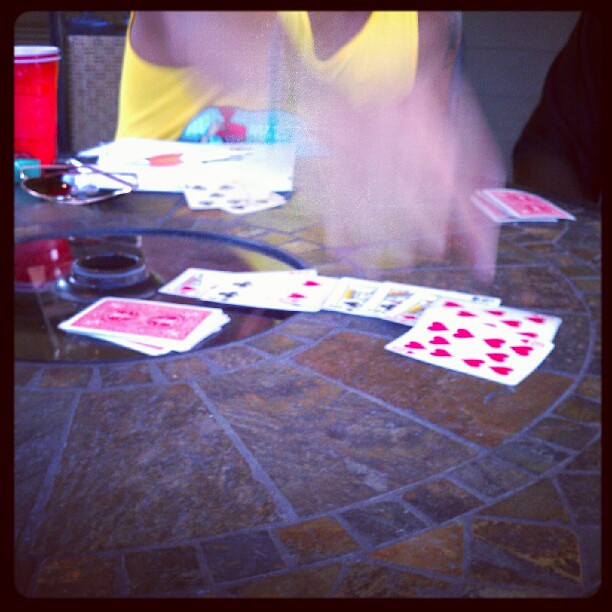A square-shaped photograph featuring a slightly blurry depiction of a card game in progress. The image is framed by a black border and centers on a round table with a dark brown and red granite design laced with light brown mortar. A glass-like section occupies the left side of the table. Scattered across the table are playing cards, distinguishable by their red backs with white borders. Among the visible cards, a king and queen of hearts stand out, while other red and black cards remain indistinct due to the blur. Two separate stacks of face-down cards are placed on the left and right edges of the table. 

In the background, characterized by indistinct gray and black tones possibly depicting a room or building, minimal detail is observed. Seated on the other side of the table is an individual with light to medium brown skin, wearing a yellow tank top. To the left of the person, a red plastic cup and a pair of black sunglasses lie face down on the table. The person’s hands are capturing mid-movement above the cards, contributing to the overall blur. Text on some of the cards is visible but remains unreadable from this perspective.